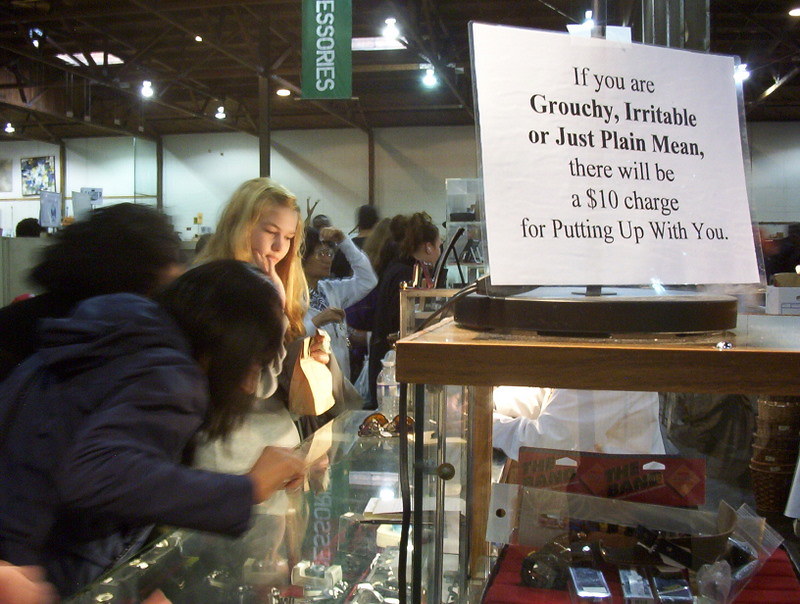This photograph captures the hustle and bustle of a crowded store, possibly an antiques show or a shop with a warehouse feel. Dominating the ceiling is a large blue sign, partially cut off, suggesting it reads “accessories.” The left side of the image showcases a glass display case containing various products, possibly jewelry or watches, observable through the presence of a blonde girl and two other women intently examining its contents. To the right, a wooden shelf houses a selection of items, including cell phones, with a humorous sign perched atop it stating, "If you are grouchy, irritable, or just plain mean, there will be a $10 charge for putting up with you." The scene is bustling, with at least a dozen people visible, underscoring the crowded and lively atmosphere of the store.